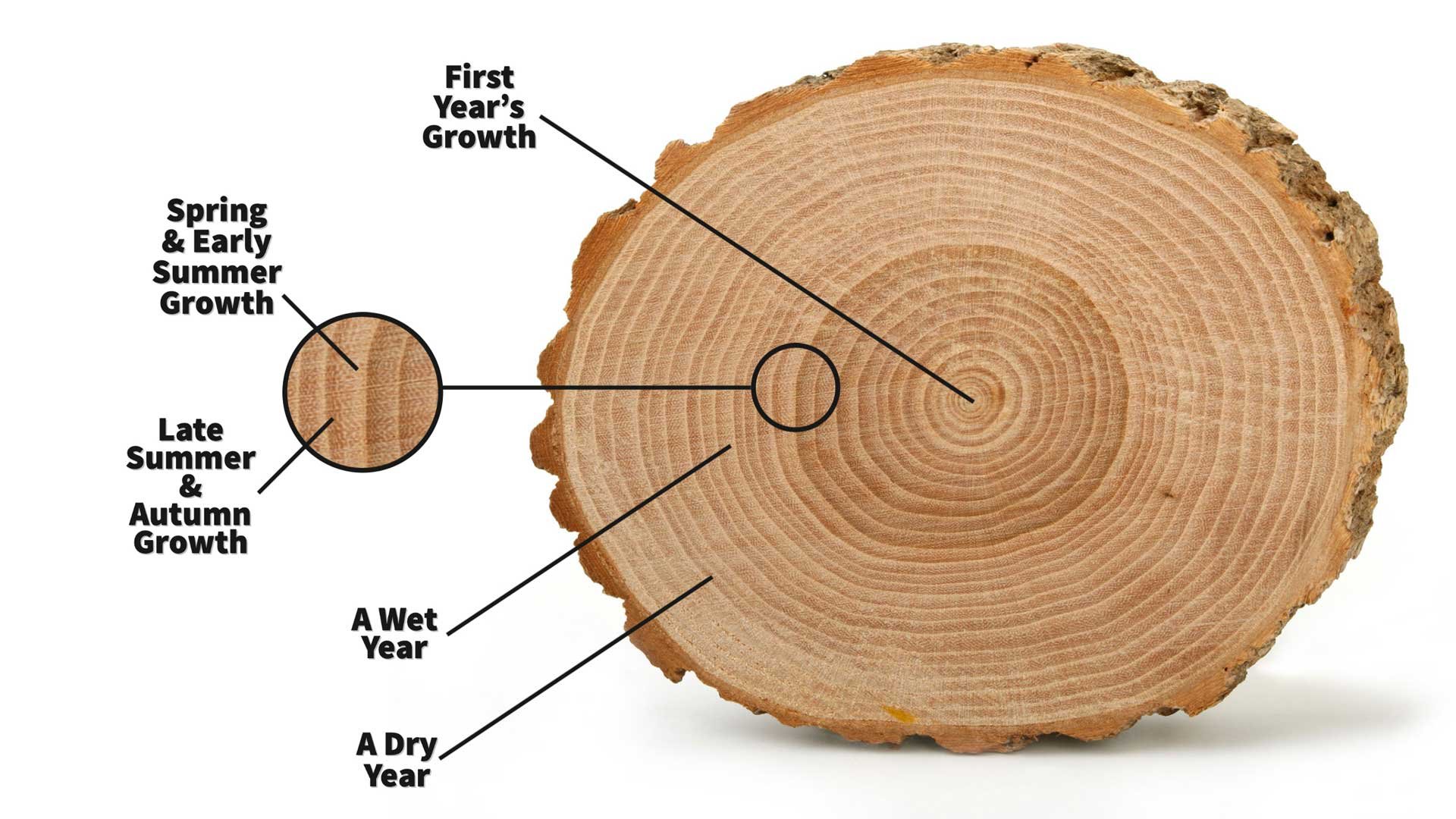This image features a detailed cutaway view of a light brown tree trunk against a white background, revealing its intricate growth rings. The tree's concentric rings vary in color from light to dark brown, signifying different periods of growth, all bordered by the rough, outer bark. To the left, black text annotates the tree's history, with lines connecting descriptions to specific ring sections. At the top, "First year's growth" points directly to the center. Below, "Spring and early summer growth" is indicated, with a magnified inset providing a closer look at these rings. Next, "Late summer and autumn growth" highlights the darker bands. Farther out, a ring marked "A wet year" shows a thicker, lighter hue, while "A dry year" points to a thinner ring closer to the bark, illustrating varying annual growth conditions.